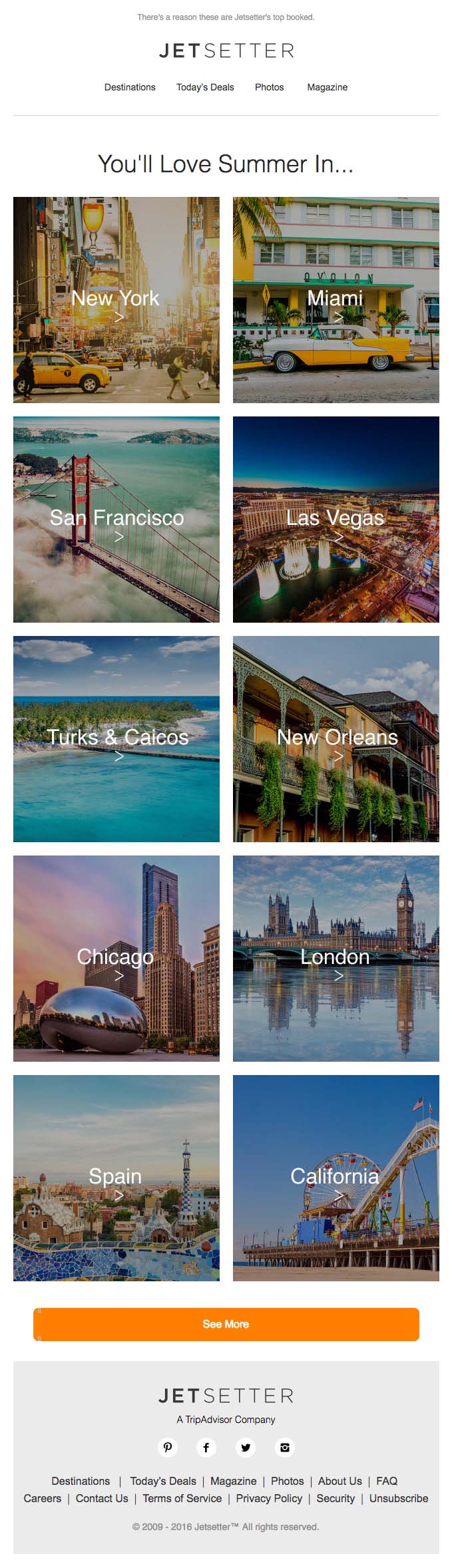This portrait-oriented screenshot appears to be captured from a mobile device, showcasing a section of the website "JETSTHER." The site has a clean, user-friendly interface characterized by a distinct header and navigation bar. 

The header consists of a subtle slogan or motto positioned above the main site logo, which is styled in all capital letters with "JETS" bolded in dark gray text, enhancing its prominence. Below the logo is a slim, light gray-bordered navigation bar, dividing it from the main content. The navigation bar includes several links, arranged as follows: the first link starts with the letter 'D,' though its full text is indistinct; the subsequent links are "Today's Deals," "Photos," and "Magazine."

The main body of the website features an engaging section titled "You'll Love Summer In..." followed by a grid of ten images that serve as links. These images are organized in a 2x5 layout (two rows of five images each), showcasing various desirable travel destinations. Each image is labeled with white text indicating the location it represents: New York, Miami, San Francisco, Las Vegas, Turks and Caicos, New Orleans, Chicago, London, Spain, and California.

Below these images is an inviting orange button labeled "Show More." The footer of the site reiterates the site logo and includes the tagline "A Trip Advisor Company." This is followed by several social media icons, providing quick access to the site’s social media profiles, and a smaller secondary footer with additional buttons for further navigation or information.